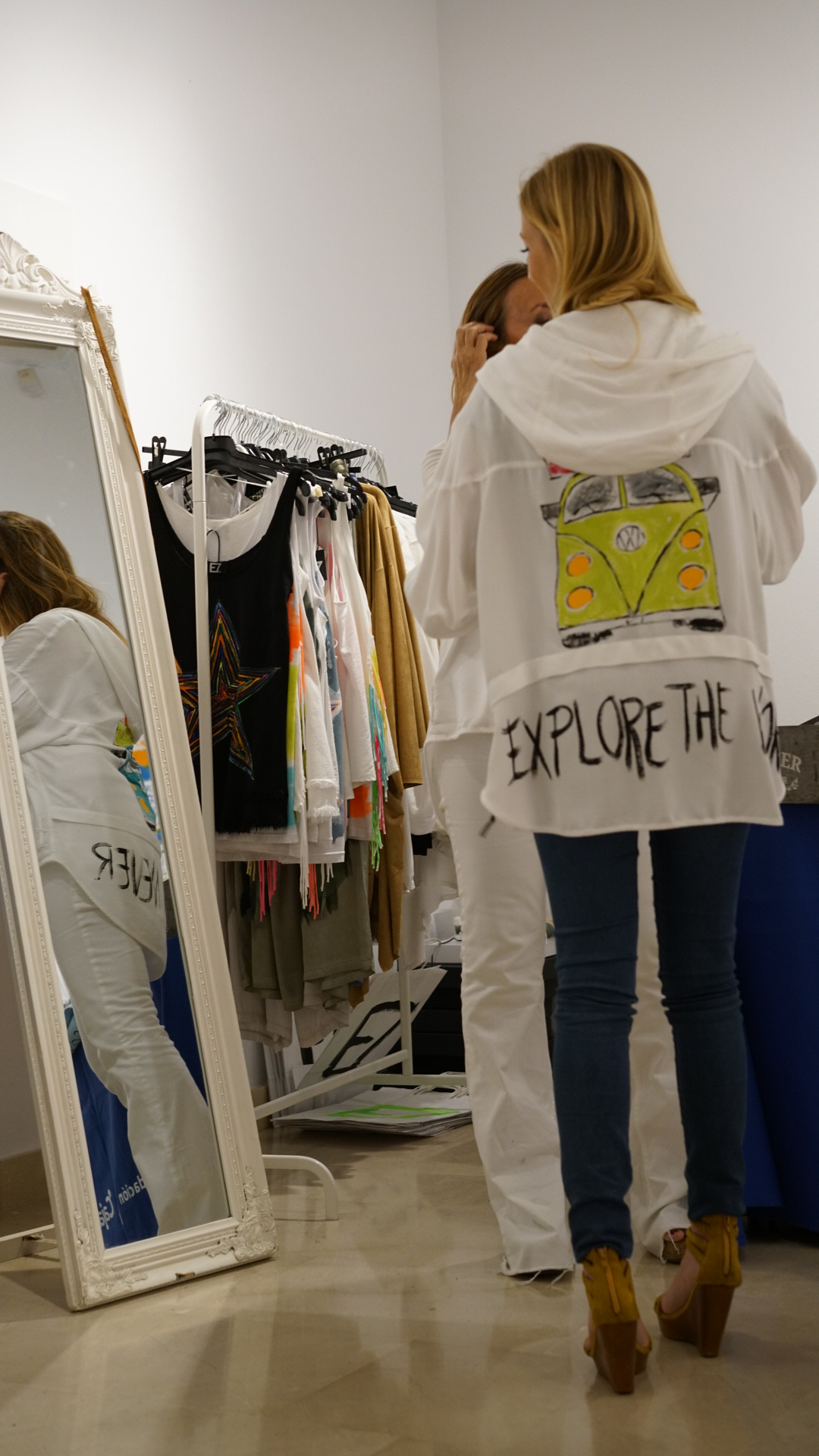In this indoor image, we observe a scene set on a tan linoleum floor. Dominating the center of the composition are a woman, likely a mother, and her daughter. The woman, who is blonde and dressed in jeans paired with high-heeled boots, is trying on a jacket inscribed with "Explore the World" alongside a picture of a VW bus. The girl appears to be looking into a tall stand-up mirror situated to the left of the frame. Surrounding them, off to the right, is a coat rack densely packed with various shirts and garments. The walls in the background are a solid white color, providing a stark contrast to the vibrant hues present in the scene, including shades of blue, black, green, orange, and red. The setting, which resembles a flea market, is devoid of any readable text and does not indicate the time of day. The overall composition highlights the centralized position of the two figures amidst the scattered objects around them.